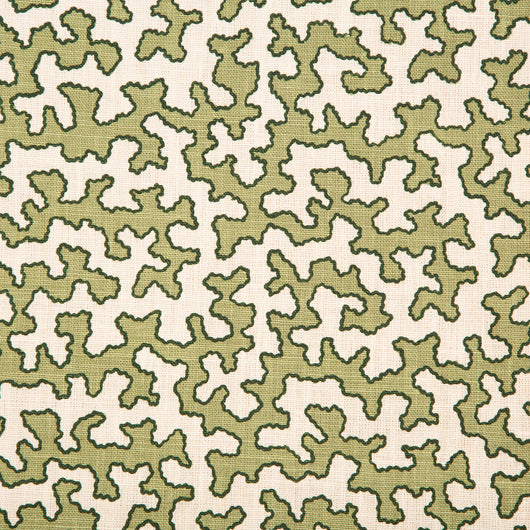This square image showcases a close-up of a textured fabric with a light tan background. The fabric is adorned with various abstract green shapes that resemble puzzle pieces or a cheetah print pattern, each outlined in dark green or black. The shapes are scattered across the fabric, allowing the light tan background to peek through. This design doesn’t form any recognizable pattern and appears random and maze-like. The cloth's texture is clear, and the image is entirely focused on the fabric, with no borders framing the square photograph.